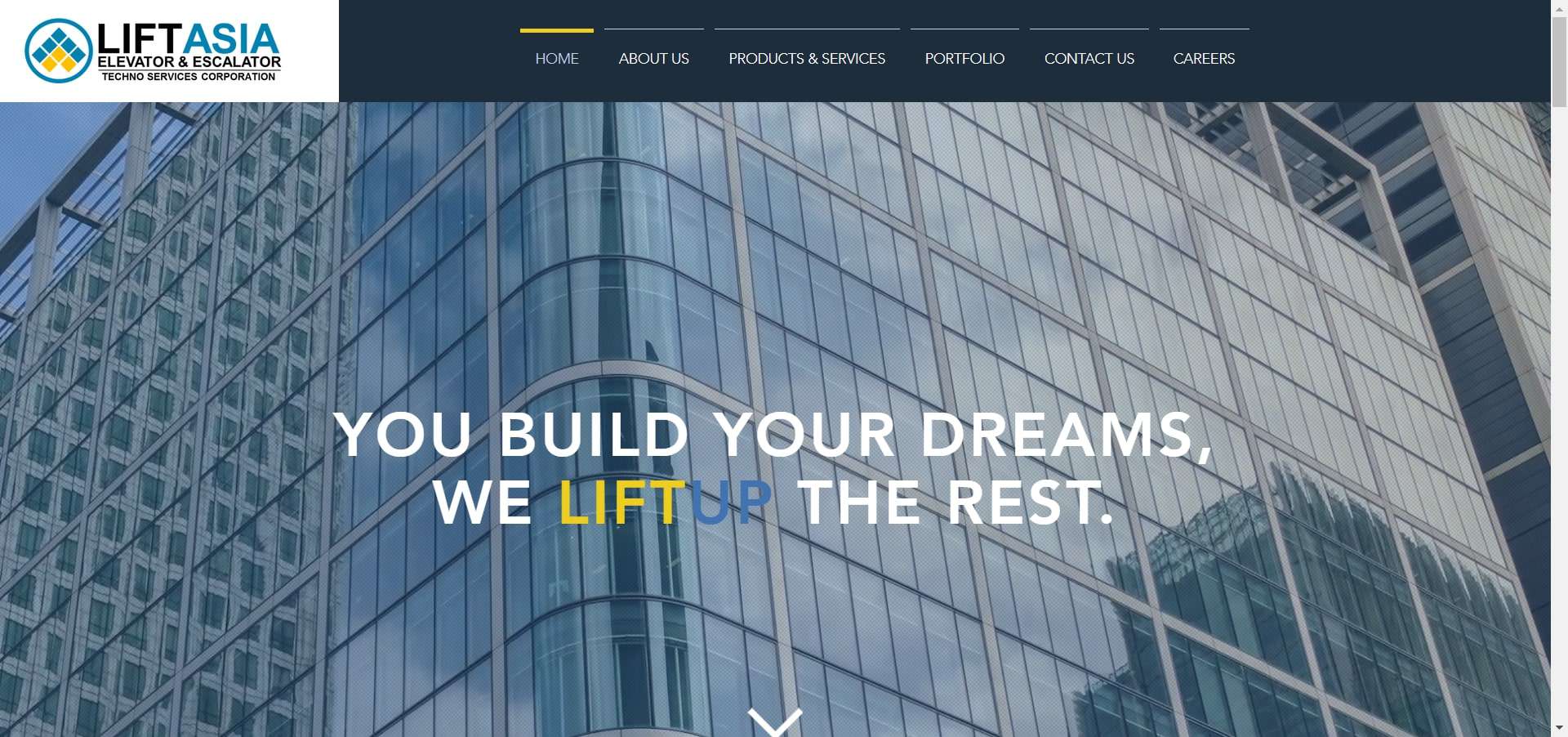This screenshot captures the home page of the "Lyft Asia" website. At the top left corner, the brand name "Lyft Asia" is prominently displayed, with the word "Asia" in blue. Directly beneath it, the tagline "Elevator and Escalator" appears in black, underlined, and followed by the smaller text "Techno Services Corporation." Adjacent to this branding, on the left, is the company’s logo: a circle featuring a pattern of interlocking squares in blue and yellow.

On the right side of the header are the website's navigation subheadings: "Home," "About Us," "Products and Services," "Portfolio," "Contact Us," and "Careers." A yellow bar above the "Home" subheading indicates that the current view is the home page.

Below the navigation bar, the entire subheading section transitions into a large banner image depicting a skyscraper with at least ten floors. The skyscraper features predominantly glass windows with metal framing, and it stands against a clear sky. Another building is visible to the right, and the reflection of an adjacent glass skyscraper is also noticeable on the primary building’s surface. 

The picture itself is slightly dimmed to enhance the visibility of prominent text overlaid on it. The text reads, "You build your dreams. We lift up the rest." The phrase is in white, except for the words "lift up," which are highlighted in yellow and blue, respectively, to emphasize the core message.